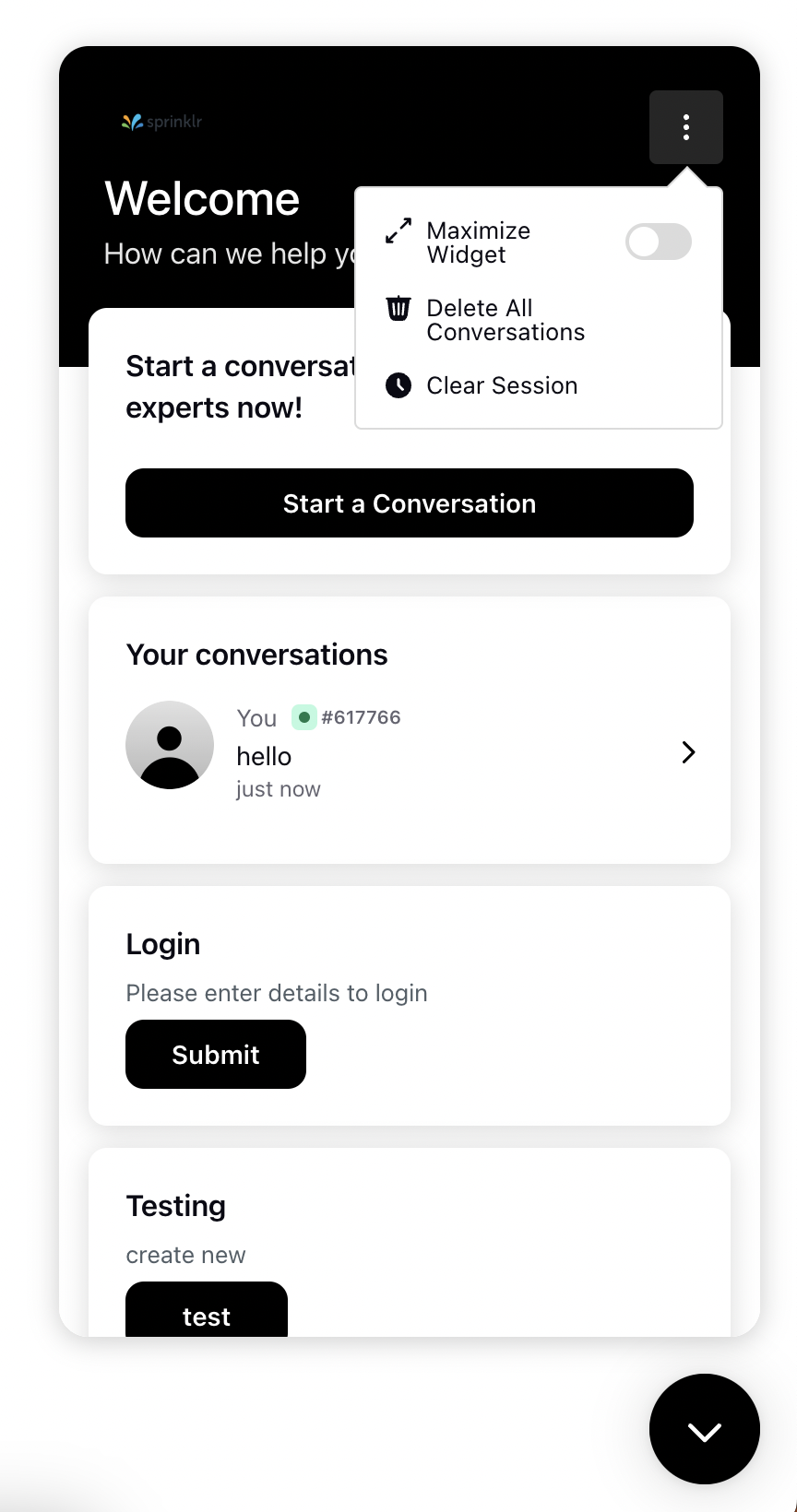This is a detailed screenshot of a mobile phone screen displaying the "Sprinklr" app interface. At the top, there is a prominent black rectangle housing the app’s header. In the upper left corner of the header, there’s a colorful plant logo resembling a sapling with four leaves – the right side is red, and the left side is blue. Next to the logo, the app's name "Sprinklr" is displayed in text.

In the upper right corner of the black rectangle, there is a small gray square with three vertical white dots, indicating a menu. A white chat bubble is seen emerging from this square, showing a pop-up menu. The first option in the menu displays an icon of two diagonal arrows with the text "Maximize widget" next to it in black font. Below that is a trash can icon with the label "Delete all conversations" to its right. The third option is marked with a clock icon and the text "Clear session."

Behind this semi-transparent pop-up menu, there is partly visible text at the top that reads "Start a conversation," followed by more obscured content. Below this, there is text that states "Experts now!" Below the "Experts now!" text, there is a black oval button with white font that says "Start a conversation."

Further down, there is a white rectangle featuring black text labeled "Your conversation." Beneath this heading, there is a message from the user identified as "you" with the number "617766" and a text input showing "hello."